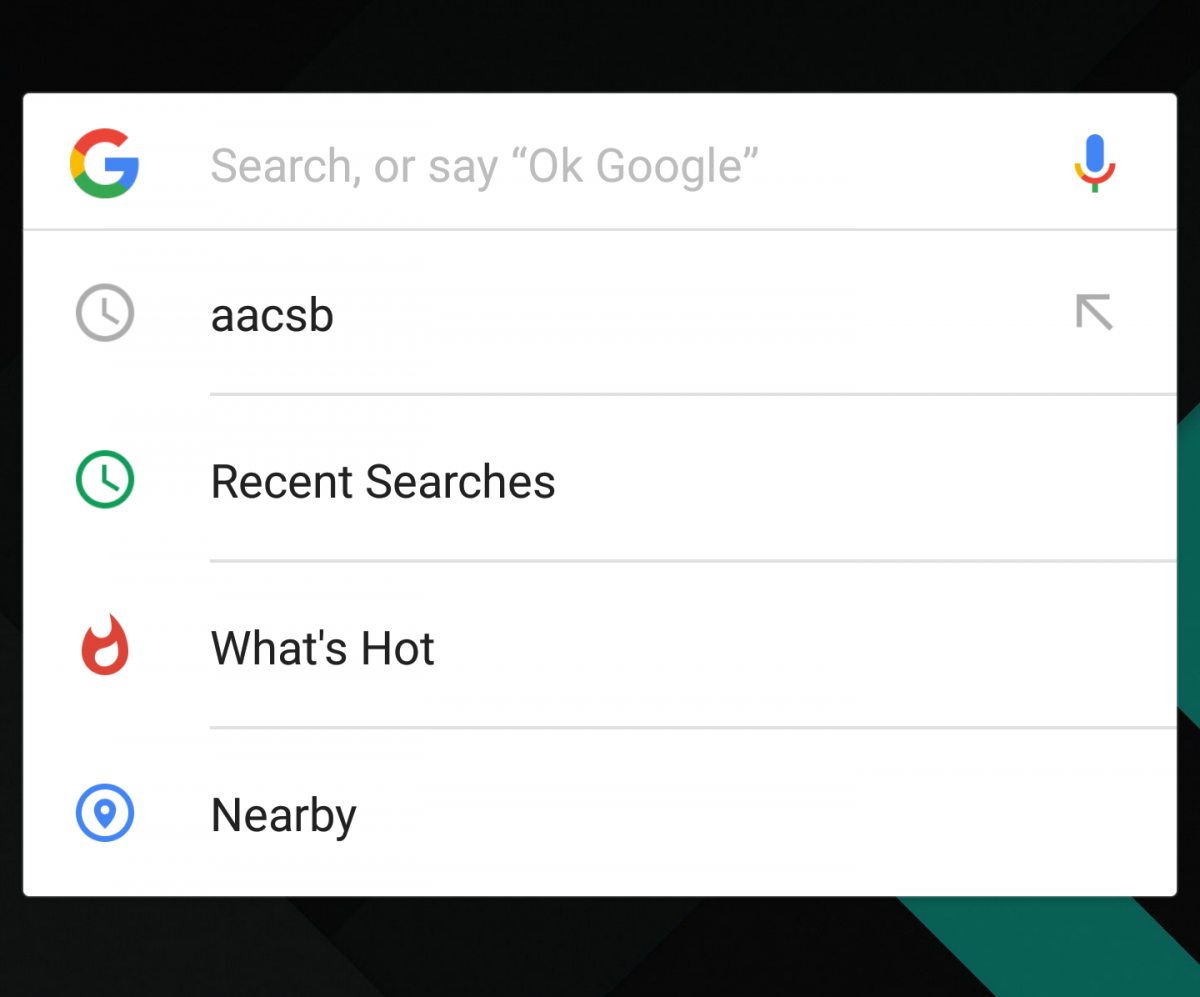The image is a square screenshot displaying a Google search interface. In the center, there is a prominent white overlay surrounded by a distinctive black and green border. The green section of the border slants diagonally towards the left at the bottom right-hand corner of the screenshot. At the top left of the white overlay, the multicolored Google logo (red, yellow, green, and blue) is clearly visible. To the right of the logo, the text reads "Search or say 'OK Google'" with a microphone icon positioned further to the right.

Beneath this header, a thin gray line spans the width of the overlay. Directly below this line, on the left, is a clock icon followed by the text "AACSB." On the right side is a diagonal arrow pointing upwards to the left. Another thin gray line separates this section from the next.

In the subsequent section, a green clock icon appears on the left with the text "Recent Searches" beside it. This is followed by another horizontal gray line. The section below features a flame icon on the left with the text "What's Hot?" This is also demarcated by a thin gray line.

Finally, at the bottom of the white overlay, there is a blue location icon on the left with the text "Nearby." Each section is clearly delineated by horizontal gray lines, organizing the various icons and corresponding texts on the interface.